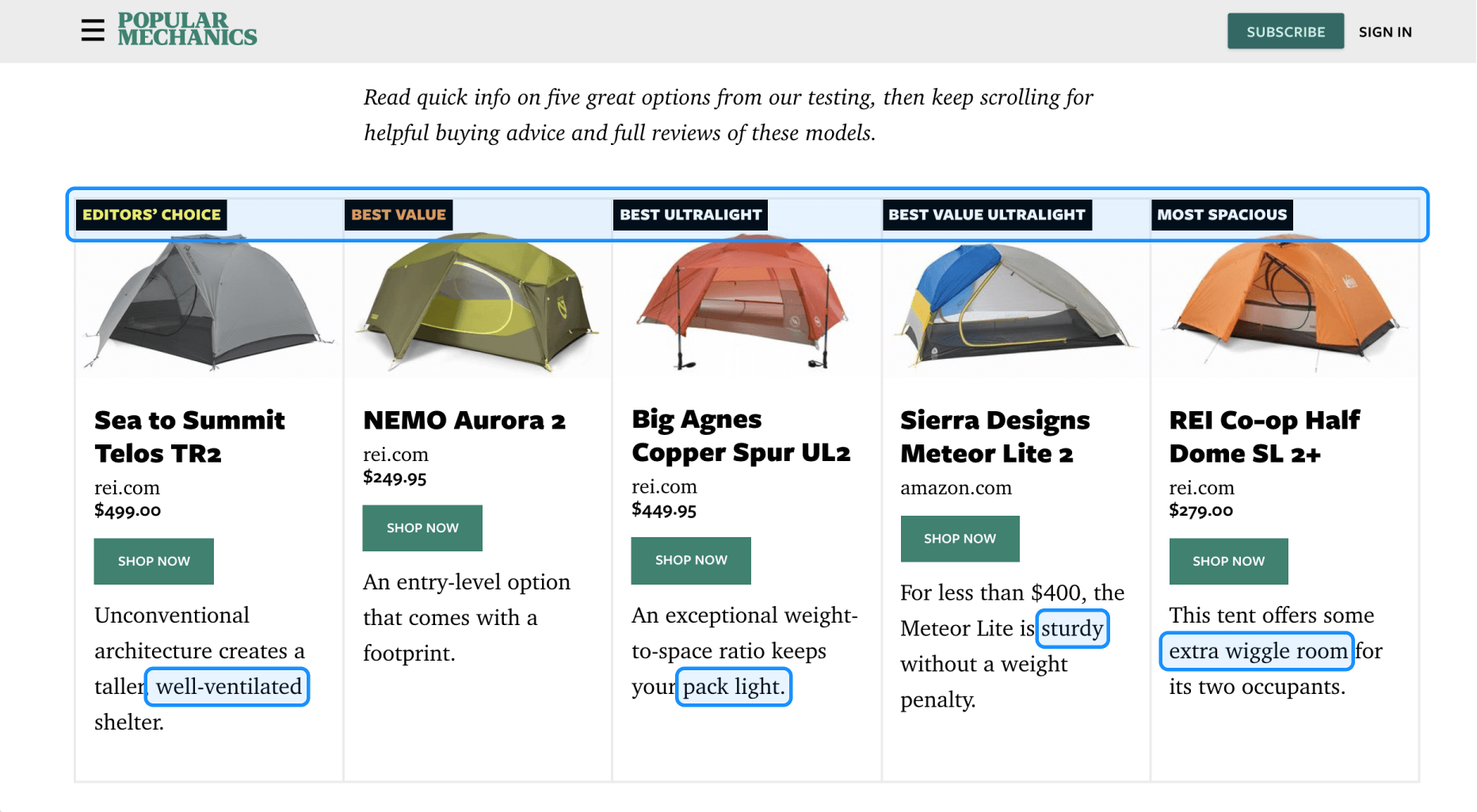**Detailed Caption:**

The image captures a section of the Popular Mechanics' website. The top header is light grey with the Popular Mechanics logo prominently displayed on the left in green. On the far right, there are two buttons: a green "Subscribe" button and a grey "Sign In" button.

Below the header, there is a text section that reads: "Read quick info on five great options from our testing, then keep scrolling for helpful buying advice and full reviews of these models." This text serves as an introduction to a detailed chart comparing different tents, rated from "Editor's Choice" to "Most Spacious."

The chart features five tents, each with a corresponding description and a "Shop Now" button. The top of the chart has tags with a black background and text in various colors, all encased in blue boxes.

1. **Editor's Choice**: Sea to Summit Telos TR2 Tent - $499 from REI.com. The description highlights that the tent is well ventilated, with the phrase "well ventilated" boxed in blue. A green "Shop" button is included.

2. **Best Value**: Nemo Aurora 2 - $249.95 from REI.com. The description emphasizes value, with a green "Shop Now" button adding convenience.

3. **Best Ultralight**: Big Agnes Copper Spur UL2 - $449.95 from REI.com. The description underscores its light packing capability, with the term "pack light" boxed in blue. A green "Shop Now" button is provided.

4. **Best Value Ultralight**: Sierra Designs Meteor Light 2 - available from Amazon.com. Its sturdiness is noted, with the word "sturdy" boxed in blue. A green "Shop Now" button is available.

5. **Most Spacious**: REI Co-op Half Dome SL2 Plus - $279 from REI.com. The description highlights the tent's extra space, with "extra wiggle room" boxed in blue. A green "Shop Now" button is accessible.

The image effectively conveys the detailed structure of the website, showcasing both user functionality and comprehensive tent reviews.